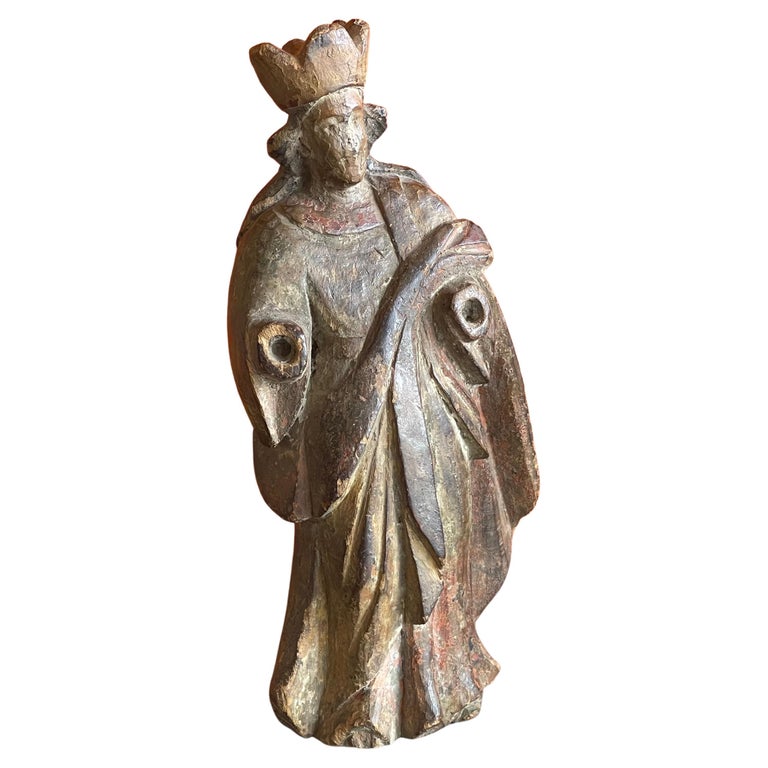This image depicts a close-up view of an ancient, detailed statue believed to represent a religious figure, possibly a priest or king. The statue is crafted from very dark wood or stone and exhibits significant aging with numerous dents and scrapes adorning its surface. The facial features are highly worn, with the nose and mouth almost entirely faded, leaving only the outline of the eyes still discernible. The figure wears a tall crown and has poofy hair styled around the ears, reminiscent of fashion from the 16th to 17th centuries. Despite the absence of its arms, with only two holes remaining where they were once attached, the intricate clothing remains intact. The figure is adorned in collared robes that wrap around its body, draped over a missing right forearm, and complemented by a flowing cape that extends to the floor, concealing any view of the feet. No inscriptions are visible on the statue, leaving its exact identity and origin open to interpretation.